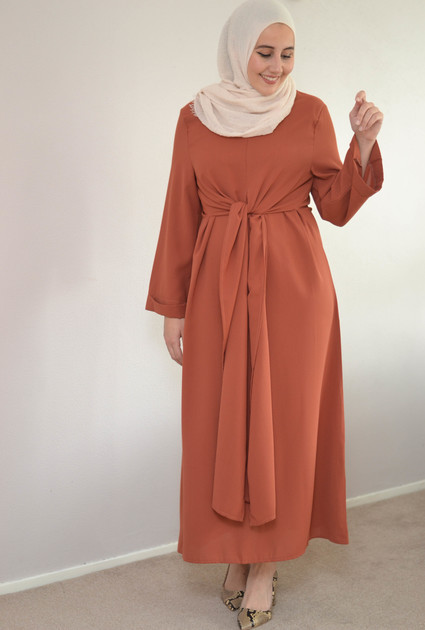The image is a color photograph of a woman standing indoors on a cream-colored carpet, slightly off-center to the right against a completely white wall. She is wearing a long-sleeved, ankle-length dress in a rich orangey-red hue. The dress features a sash or tie around her waist that drapes nearly to the hem. Her head is wrapped in a beige, scarf-like head covering that envelops her head and neck, with the remaining fabric falling behind her. She has dark black eyebrows and eyelashes, with a complexion that suggests she might be Caucasian or Middle Eastern. She is smiling and looking down, revealing her white teeth, while her left arm is raised above her shoulder and her right hand rests by her side. She completes her outfit with high heel shoes that have a snakeskin pattern.